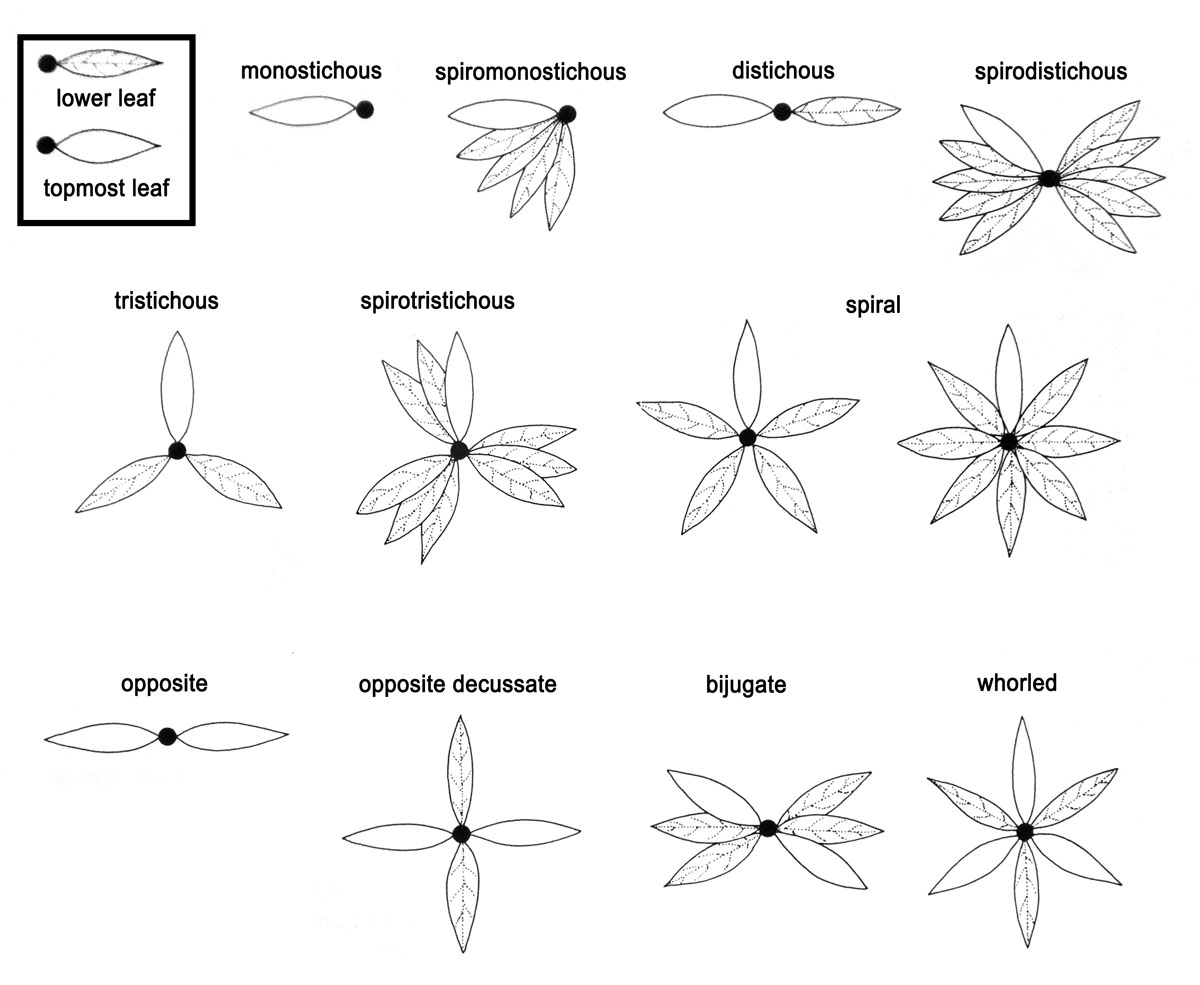This black and white digital line drawing serves as an informational poster about different types of leaves and their arrangements, set against a white background. The upper left corner features a box with illustrations labeled as "lower leaf" and "topmost leaf." The lower leaf image shows intricate vein patterns, while the topmost leaf is blank. Below this key, the main section is organized into three rows, each containing four labeled examples of leaf arrangements, namely: spiral, opposite, whorled, monostichous, spiro-monostichous, tristichous, bijugate, succinate, diastichous, and spirodichous. Some illustrations show complete leaves, while others depict partial structures. This detailed, monochromatic illustration seems ideal for those interested in botanical studies or plant identification.